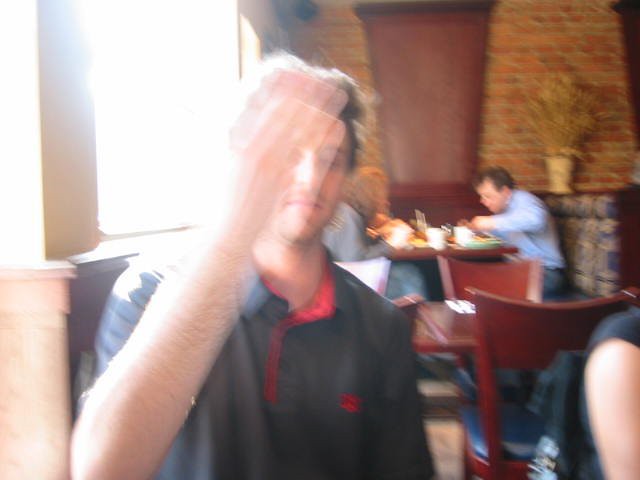This photograph captures a dynamic scene inside a well-lit restaurant dining area. Central to the image is a man with short brown hair, seemingly waving his hand in front of his face, creating a pronounced motion blur. He is dressed in a gray polo shirt with red trim and a small red emblem on the left side. Due to the blur, the details of his hand are indistinguishable. Directly behind him, a large window allows natural light to flood the scene, which adds a bright white glow to the background. The dining area features brown or brownish-burgundy chairs, and to the man's right, there is a cropped figure in a sleeveless black shirt. In the background, a booth by a brick wall is occupied by a man and a woman, engaged in their meal. The bottom right of the image reveals part of another person’s arm in a black t-shirt, adding to the sense of bustling activity.